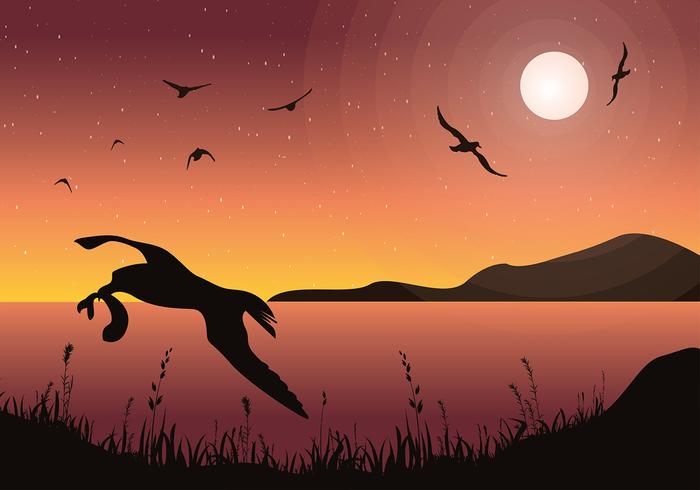A vivid painting depicts an array of silhouetted birds flying over a reddish-orange lake, framed by subtle mountains in the distance. The sky transitions from deep red at the top, gradually fading into vibrant oranges and lighter peach hues near the horizon, eventually meeting the silhouette of a distant mountain. A prominent white moon is situated in the upper right corner, radiating larger concentric circles outward, surrounded by sprinkled stars. Two birds with outstretched wings circle around the moon, while a group of four birds, positioned slightly to the left, follows. Among these four, the two birds at the top have their wings fully expanded, the middle one has its wings at its side, and the smaller ones in the distance also have their wings at their sides. In the foreground, above the dark silhouette of foliage and shoreline, another bird with outstretched wings can be seen, holding a fish in its beak. The lake below mirrors the sky's colors, blending red and orange beautifully, complementing the layers of detail throughout the scene.